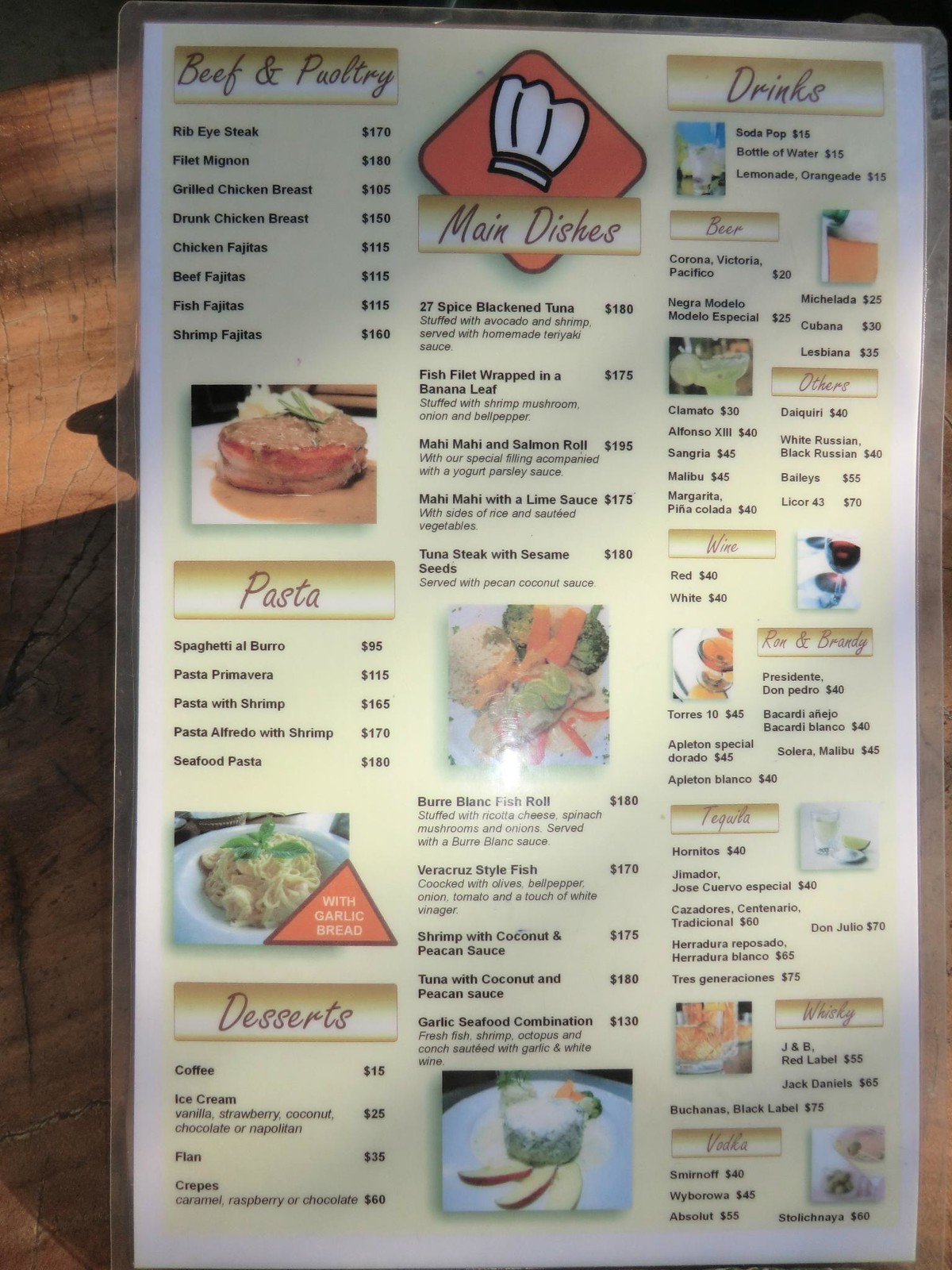This image captures a laminated menu laid flat on a wood-grain table, photographed with a standard camera. The menu itself is a single, full sheet, organized into various sections. 

In the top left corner, there's the "Beef and Poultry" section, followed by a "Pasta" section just below it. An image of an entrée featuring abundant pasta and meatballs dominates this area, with an icon indicating it includes garlic. Below these sections, there is a "Desserts" category.

At the center of the menu, there’s a red diamond backdrop featuring a chef's hat icon. This central section highlights the main dishes, numbered one through five, accompanied by a picture of one such dish. The menu then continues listing main dishes six through ten, beside another photograph which appears to show sushi and apple slices artfully arranged.

The far right of the menu is dedicated entirely to drinks, meticulously listed from top to bottom.

The combination of images and organized sections offers a comprehensive overview of the menu's offerings, making it easy for diners to navigate and choose their desired items.